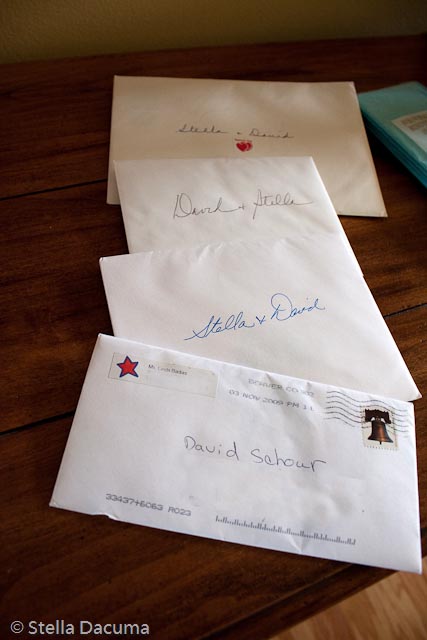The image is a color photograph, oriented upright like a page, depicting a dark wooden table made of three wide planks. On the table, there are four envelopes.

1. **Foreground Envelope:** The most prominent envelope is addressed to David Schour. It has a Liberty Bell postage stamp with a cancellation mark, suggesting it went through the mail. There is also a printed return address label with a red star, although the return address and the recipient's address appear to be whited out or digitally removed.

2. **Second Envelope:** Laying behind the first, there is a square-shaped envelope addressed to Stella and David, handwritten in blue ballpoint pen.

3. **Third Envelope:** Another envelope partially visible behind the second one is addressed to David and Stella, written in black pen. The handwriting on both this and the previous envelope suggests they were written by the same person. 

4. **Rear Envelope:** The fourth envelope, positioned flat on the table, is addressed to Stella and David and features a small red heart or apple sticker underneath the names.

In the upper right corner of the image, there is an aqua-colored object, possibly a small travel pack of Kleenex, with a visible but indistinct label. The scene is complemented by a lighter wooden floor at the bottom of the image. Additionally, the bottom left corner of the image bears a watermark in white font that reads "Stella Dacuma."

The details collectively paint a scene of thoughtfully addressed and possibly hand-delivered envelopes, carefully arranged on a wooden surface.